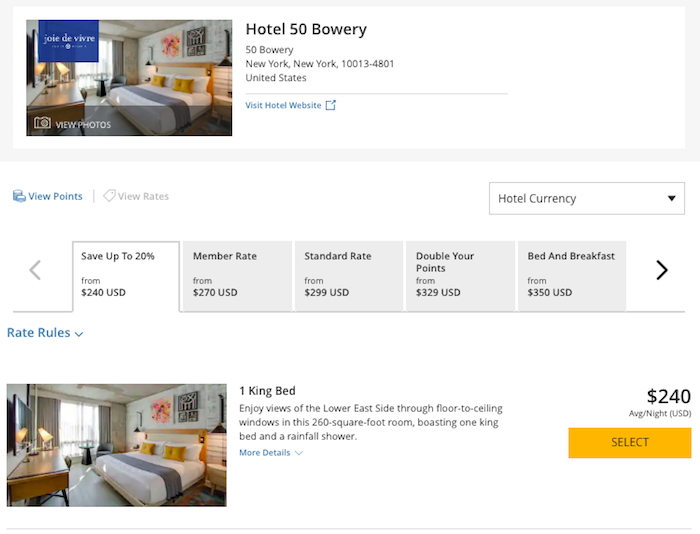The image is a screenshot of the website for Hotel 50 Bowery located in New York City. On the left side of the image, there's a photograph of one of the hotel's bedrooms. The room features a large king-size bed adorned with vibrant yellow pillows, positioned against a backdrop of tasteful modern bedroom furniture. The room has a large window allowing natural light to pour in, and it is furnished with chairs, a table, and elegantly draped curtains. 

Above the bedroom image, there's a text that reads "view photos" and "joie de vivre," suggesting a focus on the delight of living well. Below the image, a section in blue text titled "viewpoints" is highlighted, indicating different pricing options for booking a room. 

- **Save up to 20%**: Starting from $240 USD, this option is highlighted.
- **Member Rate**: From $270 USD.
- **Standard Rate**: From $299 USD.
- **Double Your Points**: From $329 USD.
- **Bed and Breakfast**: From $350 USD.

Under the selected "Save up to 20%" category, further details are provided. The room features one king bed with a description stating, "Enjoy views of the Lower East Side through floor-to-ceiling windows in this 260 square foot room, boasting one king bed and a rainfall shower." A blue text link labeled "rate rules" offers more detailed information about the rates. Additionally, there's another blue text link labeled "more details" with a downward arrow for additional information.

On the far right side of the image, in black text, the price is listed as "$240 average/night USD." Below this, there is an orange rectangular button that allows the user to select this room and move forward with the booking process.